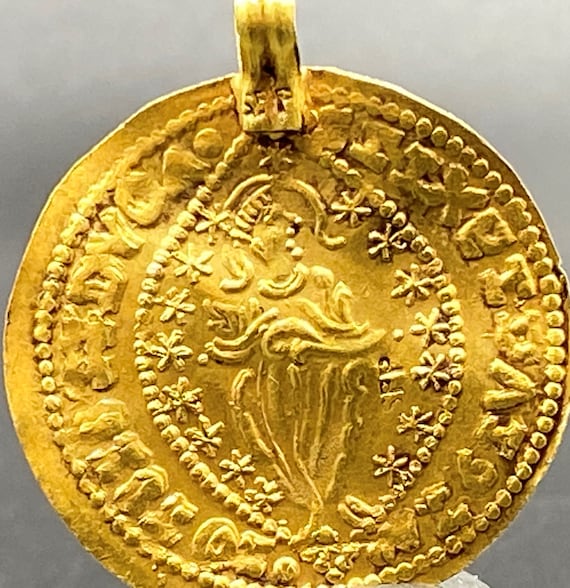This photograph features a highly detailed, ornate gold medallion-style coin, designed to be worn as a necklace due to the clasp or handle at the top. The medallion is thin and dominates the image, set against a subtly varied gray background. At the center of the medallion is an engraving of a seated woman with her knees drawn up, surrounded by star or snowflake-shaped symbols, all encircled by a ring of beads. Further out, another ring of engraved patterns and small circles forms a layered border. The coin appears to have a sequence of Roman numerals and letters, possibly initials like "S.P.P.," interwoven with intricate shell and floral patterns. The overall design is both complex and symmetrical, with each detail meticulously carved into the golden surface.